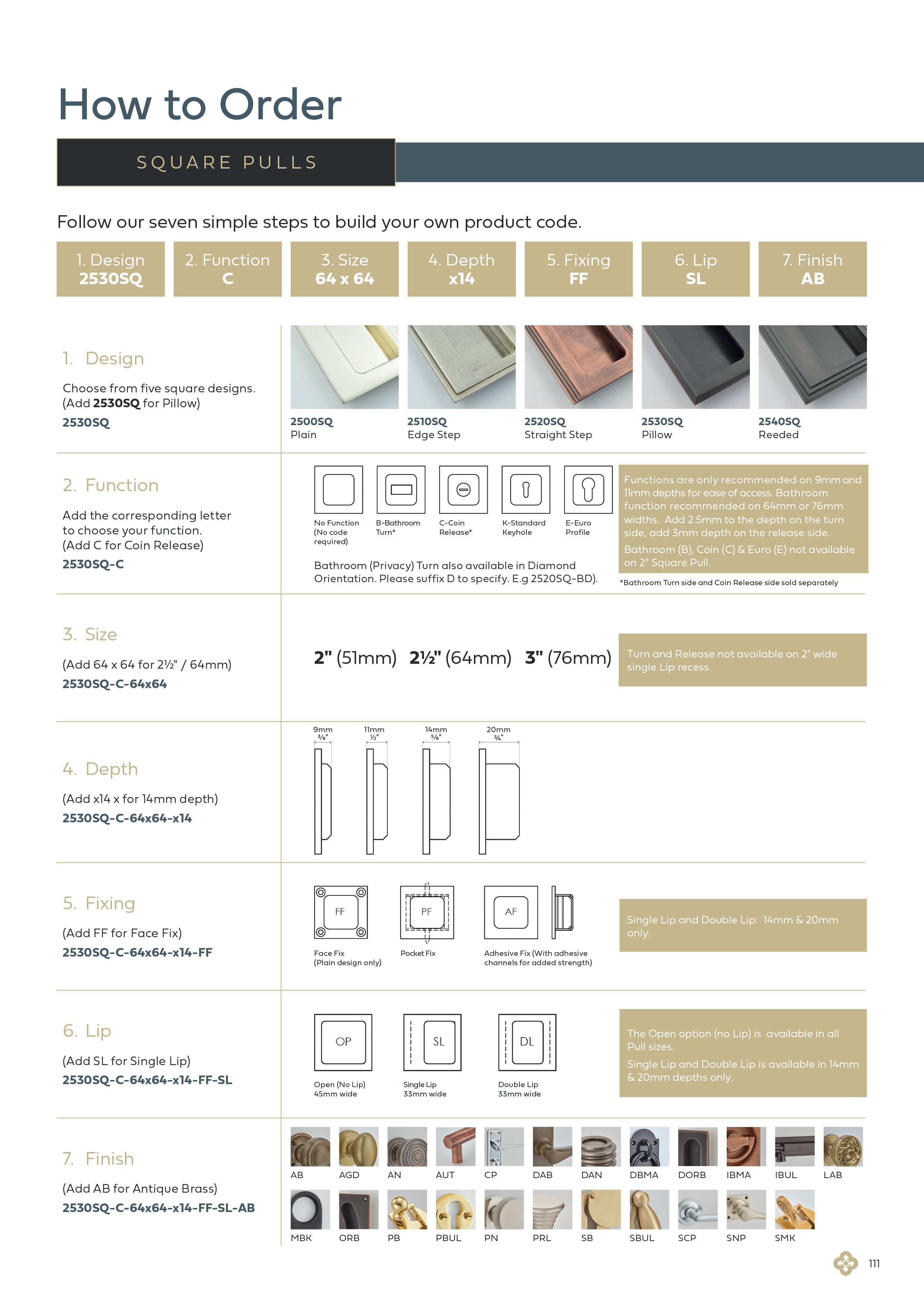The image is a detailed guide on "How to Order Square Pools," prominently labeled in the top left-hand corner. This comprehensive guide is structured to assist users in customizing their square pools through a step-by-step process. It features several design numbers and seven distinct categories: Design, Function, Size, Depth, Fixing, Lip, and Finish. Each category provides specific criteria to build a unique product code that corresponds to the user's requirements. The guide visually represents different examples of these square pools, which intriguingly resemble kitchen utensils. These examples are presented in a variety of colors, including white, pink, black, and gray. The entire layout of the guide is set against a clean, white background, enhancing readability and focus on the details provided.